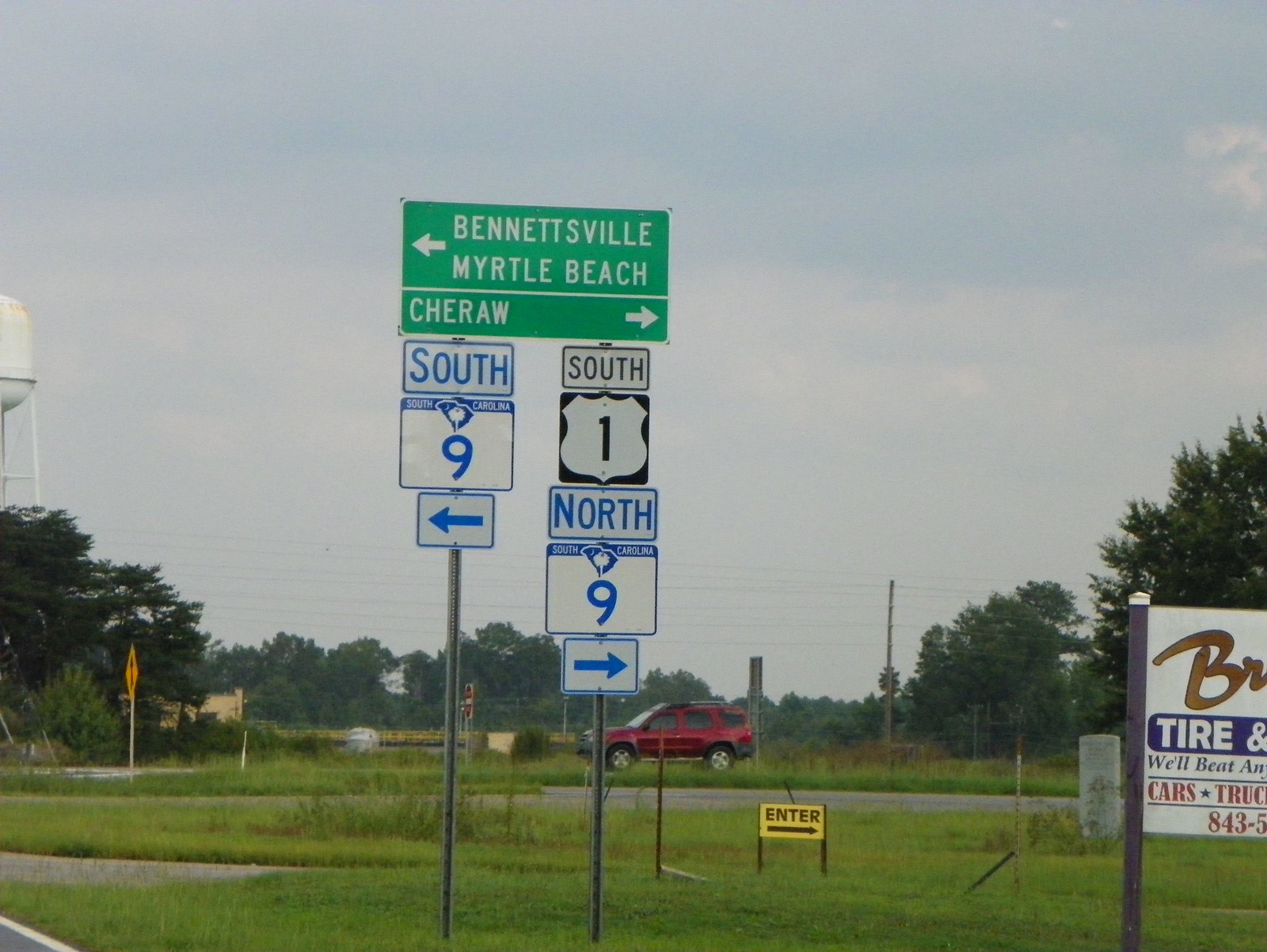In this rectangular, horizontally oriented photograph taken in a rural setting, the scene focuses on a crossroads flanked by street signs. Prominently in the center bottom of the image, multiple signs mounted on metal poles provide directional information. At the top of the pole is a green sign with white lettering that reads "Bennettsville Myrtle Beach," complemented by an arrow pointing left, indicating west. Directly beneath it, another green sign reads "Cheraw," with an arrow pointing right, indicating east.

Further down the pole, a white sign with blue print indicates "South 9," with an arrow also pointing left, directing west. Adjacent to this, a black and white sign reads, "South 1 North South Carolina 9," with an arrow pointing to the right, denoting an eastern direction. The base of the pole is surrounded by green grass, which contrasts with the metallic gray of the poles and signs.

In the lower right corner of the image, a partial sign peeks into view, displaying the words "Tire, Cars, Truck" along with the area code "843," hinting at nearby automotive services. The background reveals an open country setting, adding to the tranquil, pastoral atmosphere of the photograph.